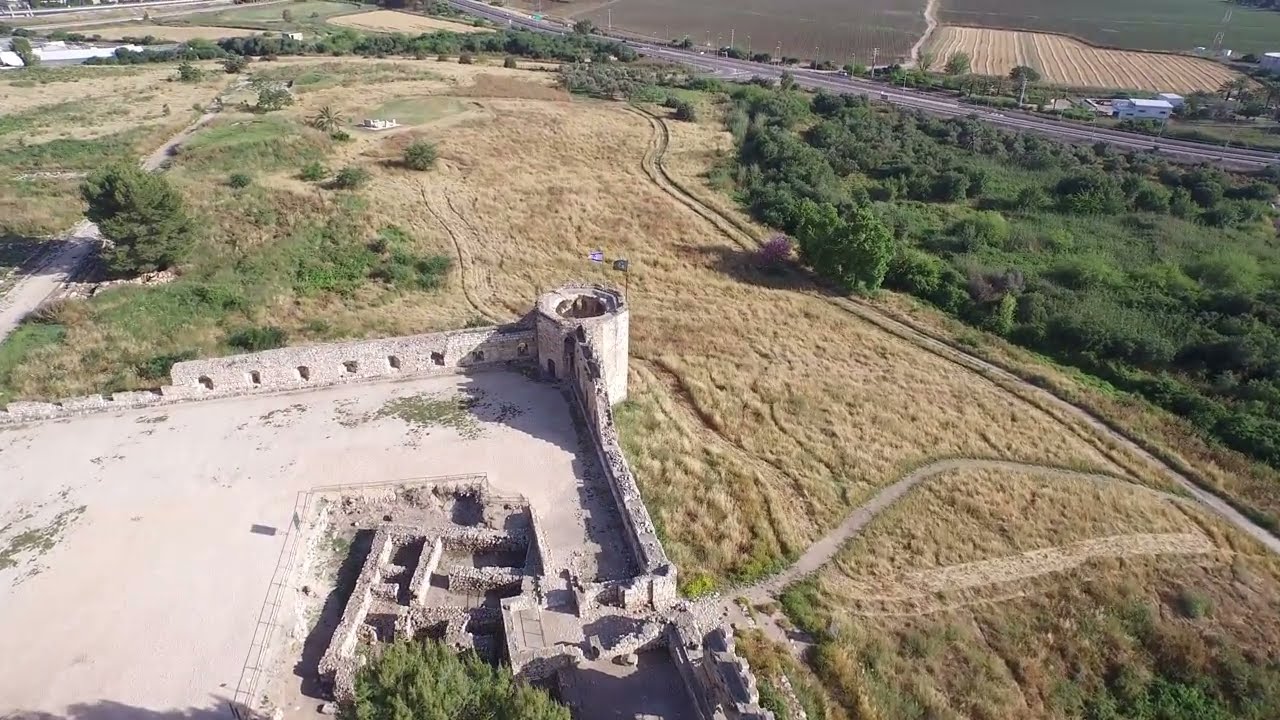An aerial view captures an expansive landscape primarily composed of yellowed, sun-scorched grass, interspersed with patches of greener grass and clusters of bushes and trees, especially to the right and left edges. In the center lies what seems to be the weathered and partially demolished cement foundation of an old castle-like structure, framed by a stone ledge. The structure, largely built from stone and brick, shows signs of heavy wear, with visible torn-down sections and an intriguing brick inlay. Adjacent to this ruin, a mowed pathway meanders through the dead grass, leading towards a distant road situated in the upper right corner, which features white lines and separates this expansive, undeveloped land from more cultivated regions. Beyond the road, additional grasslands, plowed fields of tan and yellow hues, and white-roofed houses suggest a rural, somewhat run-down area. A gray road extends from the left and curves up into the image, enhancing the sense of isolation in this open, windswept agrarian landscape.